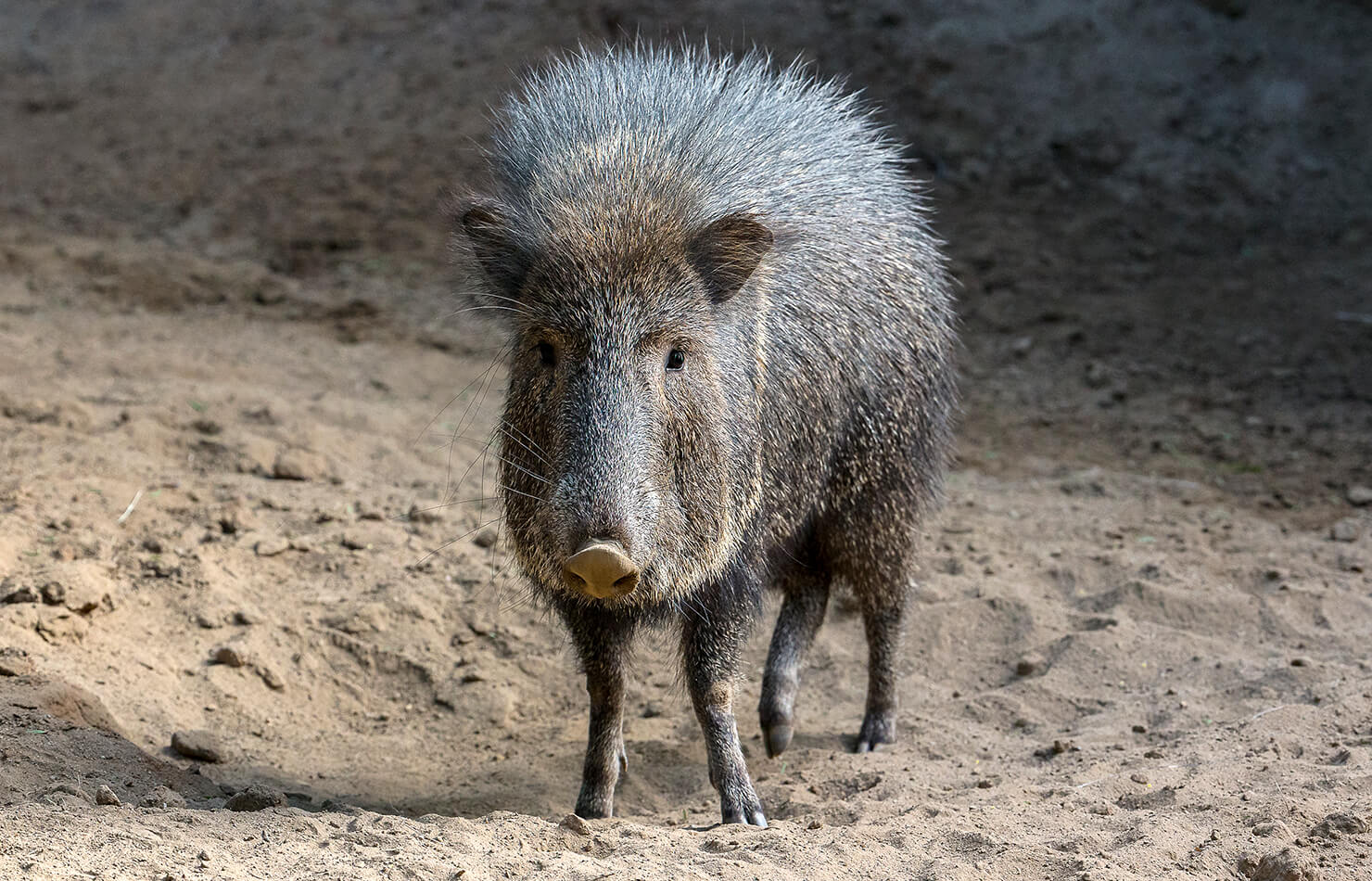This professional, full-color outdoor photograph captures a wild hog, possibly a warthog, standing in a sandy, rocky area under a bright sunlit sky. The creature has a distinctive appearance with thick, long brown hair spiking up along its back, and a face that’s more narrow and elongated than a typical pig. Its small, beady black eyes and a flat, tan snout are clearly visible, and its rugged appearance is emphasized by the dusty, rough terrain it stands on. The animal's grayish-white hair and stout but thin-legged physique underscore its rugged life in a harsh, dry environment. Staring directly into the camera, the hog seems to scrutinize the observer, adding an element of wild curiosity to the scene.